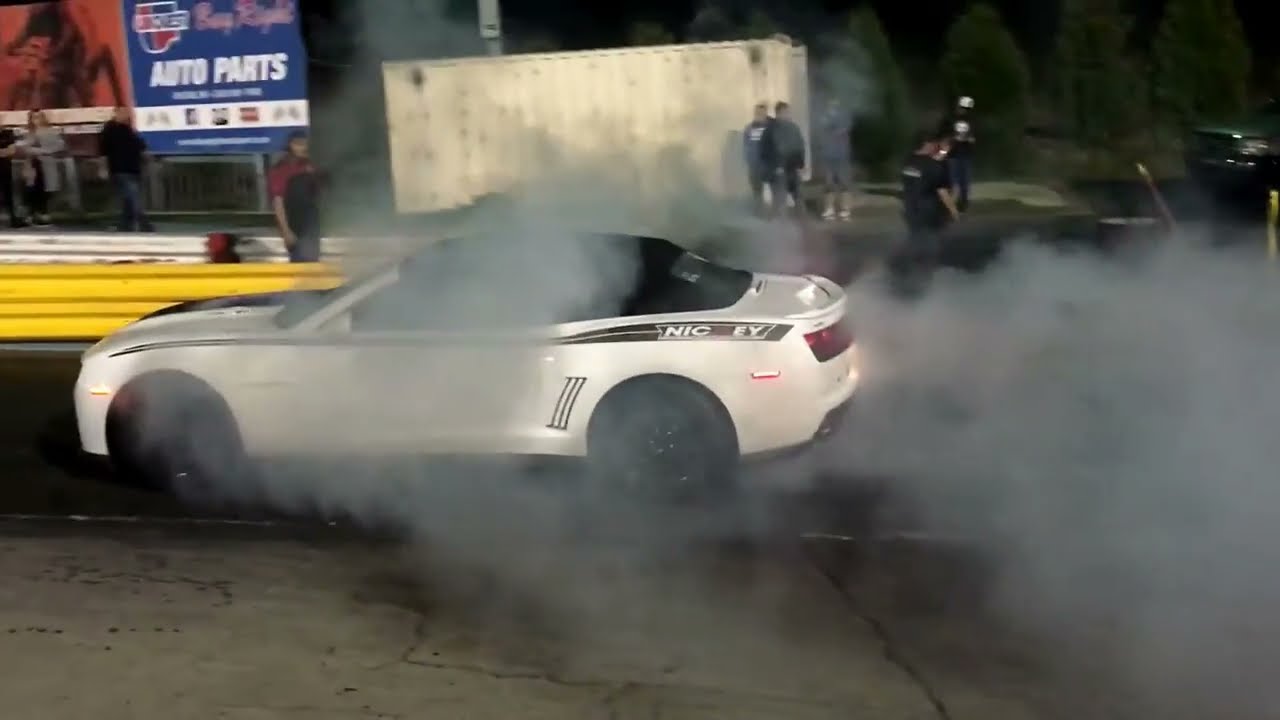The image depicts a white sports car, identified as a Mustang, engaged in what appears to be a dynamic burnout on a nighttime test track or parking lot. The car features a black roof and black rims, with white bodywork accented by a pinstripe that starts thin near the engine and widens towards the trunk. Thick smoke envelops the vehicle, emanating from its tires, suggesting high-speed wheel spinning. The Mustang, showcasing the text "N-I-C-E-Y" in white letters, is positioned slightly to the left of center.

In the background, several people, possibly spectators or technicians, stand around observing the scene. To the upper left, a blue sign advertising auto parts is visible, alongside a yellow guardrail. Central to the backdrop is a large white shipping container, with more onlookers gathered around it. A few trees are discernible in the upper right against the dark sky. The image, rich in colors such as white, black, yellow, red, blue, pink, green, brown, and gray, captures the adrenaline of a nighttime car performance event.